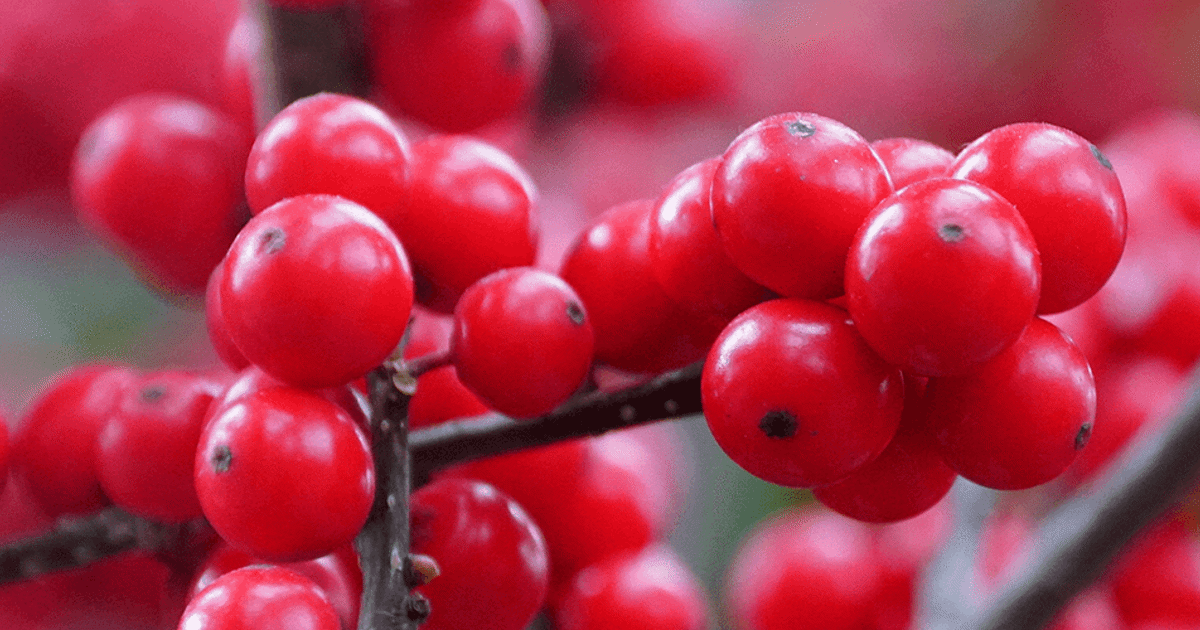The close-up image captures clusters of small, shiny red berries, approximately the size of peas, growing densely on dark, almost black, twigs and stems. The primary stem in the foreground showcases three round berries with small brown tips at their ends, while a larger branch extends across the frame featuring a prominent cluster of nine berries. Bright sunlight bathes the scene, enhancing the glossy surface of the berries and casting a vibrant sheen. The background is artistically blurred, ensuring the viewer's attention remains on the vividly detailed berries in the foreground, though additional berry clusters are visible within the soft focus. The overall composition is tightly cropped, filling the frame with the striking red and minimal green highlights, creating an intense and colorful visual impact.